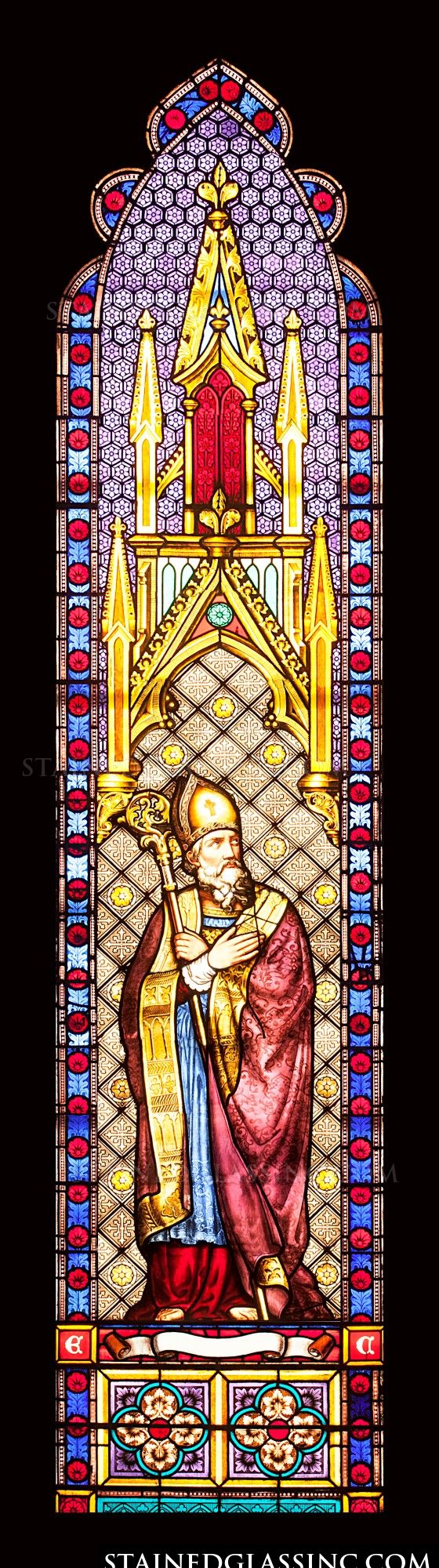This image showcases a highly detailed and vibrant stained glass window set against a solid black background to highlight its intricate designs. At the bottom, the text "stainedglassink.com" is displayed in white, indicating the creator or seller. The stained glass window features a floral pattern at the bottom, with a red-dotted center flower surrounded by yellow petals, encircled by light blue, all contained within a golden square. The window's outer perimeter is blue with red circular details. The window narrows as it ascends, eventually forming an angled, curved top. In the middle of the window, a religious figure, possibly a bishop or a saint, is depicted. He wears a gold pointed hat, red robes trimmed with gold, and a blue garment underneath a red skirt, and appears to have bare feet. Above this figure, there is a golden cathedral-like arch with pillared points. The window, abundant in vibrant hues of purple, blue, pink, yellow, gold, red, light blue, and white, stands out due to its bright and alluring colors, commonly found in Roman Catholic church settings.